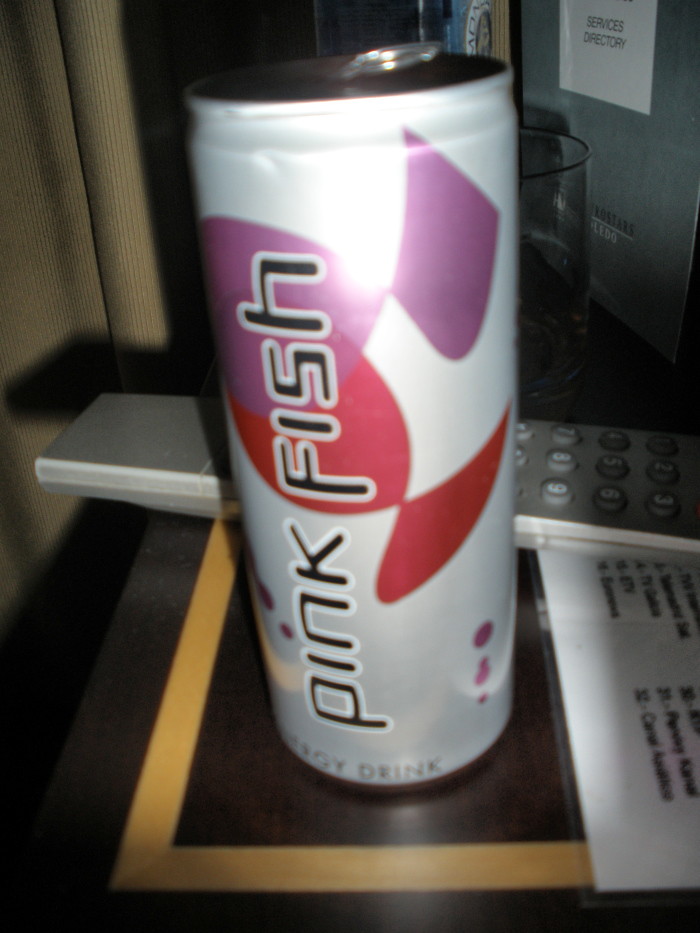The image features a tall beverage can, distinctly slimmer and shorter than a typical soda can. The can is a light gray or off-white color, adorned with pink and purple bubbly designs. Prominently displayed on its side are the words "Pink Fish" in bold black letters outlined in white. The can's silver tab and rim are visible at the top.

Behind the can, a silver long remote control is placed horizontally. This remote has numerous buttons, including gray and circular ones with white numbers. To the right of the can, there appears to be a silver or gray panel, possibly a book, standing upright. A white tag on this object reads "Services Directory."

The background of the image is relatively dark, featuring brown curtains. Other items in the image include a glass, and what appears to be a white laminated informational sheet detailing various TV channels in black letters. The scene presents a somewhat cluttered but cozy indoor setting.